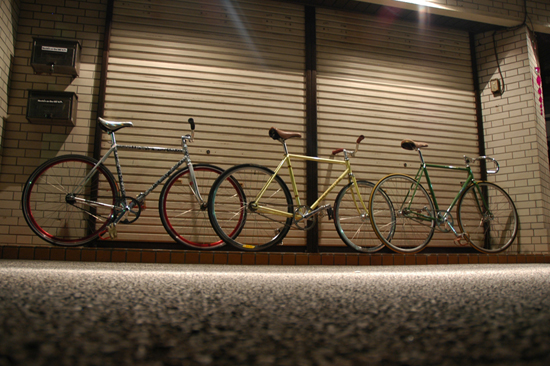This ground-level amateur photo captures three classic racing bicycles positioned in front of a white brick building with closed beige-taupe shutters, likely representing a store or garage door given the horizontal paneling and central black divider. The three bicycles, each with skinny wheels and silver pedals, stand upright without support. The bicycle on the left features a green frame with curved handlebars, the middle one has a yellow frame, and the one on the right shows a blend of silver and green with straight handlebars. The scene includes pavement with visible black and white specks at the bottom of the image. On the left side of the building's entrance, there are two black mailboxes attached to the brick wall. A light fixture is visible above the bikes, adding to the intricate details of this everyday setting.